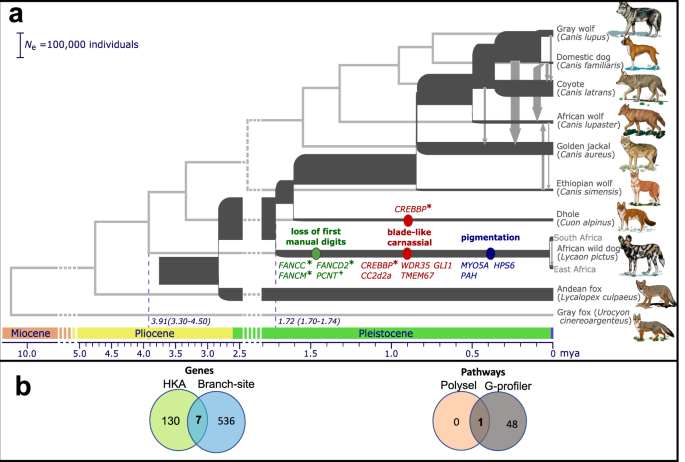The image depicts a detailed timeline with a white background in a rectangular format. In the upper left-hand corner, there is a black letter "A." Along the right side, there's a list titled "Wolf Family," featuring both images and names of various canids. The list includes the grey wolf, domestic dog, coyote, African wolf, golden jackal, Ethiopian wolf, dhole, South African fox, Indian fox, Andean fox, and grey fox. Additionally, the timeline indicates the historical presence of each species. Towards the bottom of the image, beneath the list, there is a section labeled "Genes and Pathways," which highlights genetic markers such as myosin and phylosin. Each gene is associated with the corresponding canid species, illustrating the genetic pathways and relationships among these animals.